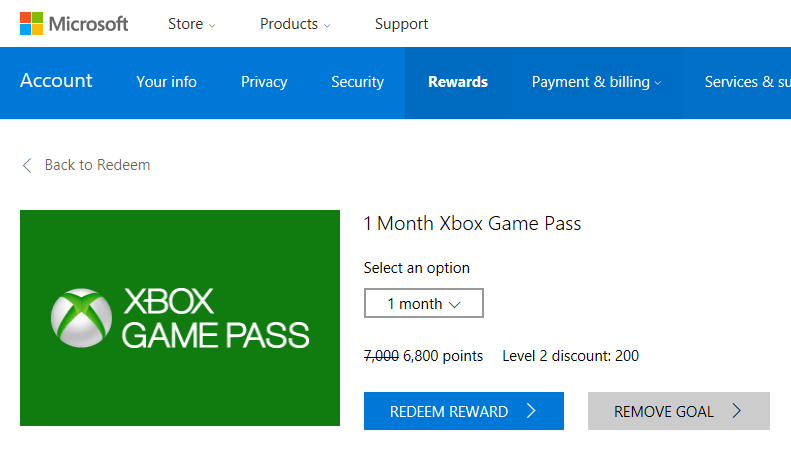The webpage is a product page on the Microsoft website. Positioned at the top left corner of the screen is the Microsoft logo, a distinctive square composed of four smaller squares in dark orange, green, sky blue, and yellow, with the word "Microsoft" appearing to the right of the logo. The central focus of the page is a product offering a one-month subscription to Xbox Game Pass. Directly below the product title, users can choose the duration of their subscription through a selection dropdown. Further down, the redeemable points for one month of Xbox Game Pass are indicated as 6,800 points. Located to the right of this point value is a notation stating "Level 2 Discount: 200," signifying that 200 points have been deducted from the standard redemption requirement.